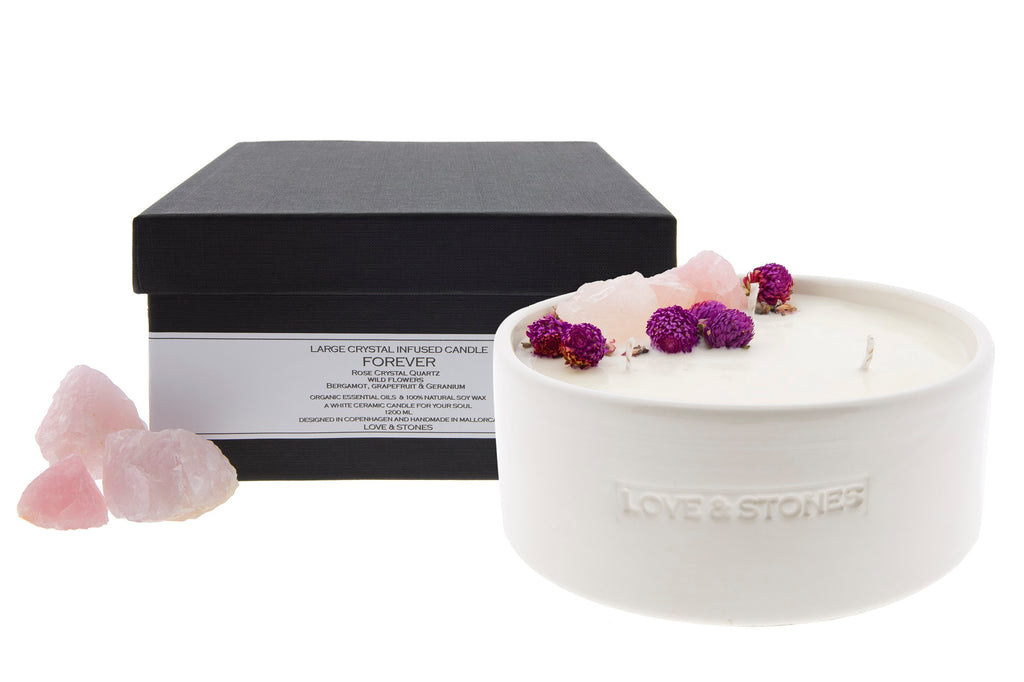The image features a detailed arrangement of a candle and its packaging, set against a seamless white background. At the forefront, there is a short white ceramic bowl labeled "Love and Stones," containing white wax with three small wicks protruding from the top. Decorative elements such as light pink crystal rocks and dark purple berries are artfully placed on the wax's surface. Positioned behind the bowl is a black cardboard box with a matching black lid, showcasing a white label reading "Large Crystal Infused Candle Labeled Forever." Three additional light pink crystal rocks adorn the corner of the box. The colors predominantly include black, white, off-white, light pink, and light purple, creating a harmonious and visually appealing composition.